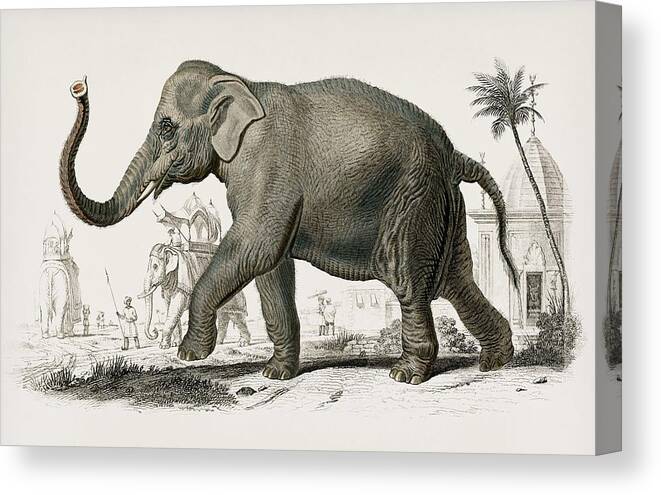The image is a detailed pencil drawing on a canvas print, noticeable by its approximately 2-inch thickness with a full wrap extending onto the sides. Dominating the scene is an old, dark grey-skinned elephant walking to the left, its trunk raised and one front leg lifted mid-step. The canvas background is predominantly white, which highlights the rich details of the elephant. In the backdrop, there is a cone-shaped temple suggesting an Indian landscape, with a palm tree prominently featured on the right side. Further back, another elephant is depicted carrying a carriage-like structure, typically used by royalty, and draped with a blanket that covers most of its body. A man, holding a stick or spear, walks beside this second elephant, guiding it forward. Sparse patches of grass and dirt hint at a natural ground setting, adding depth to the composition.